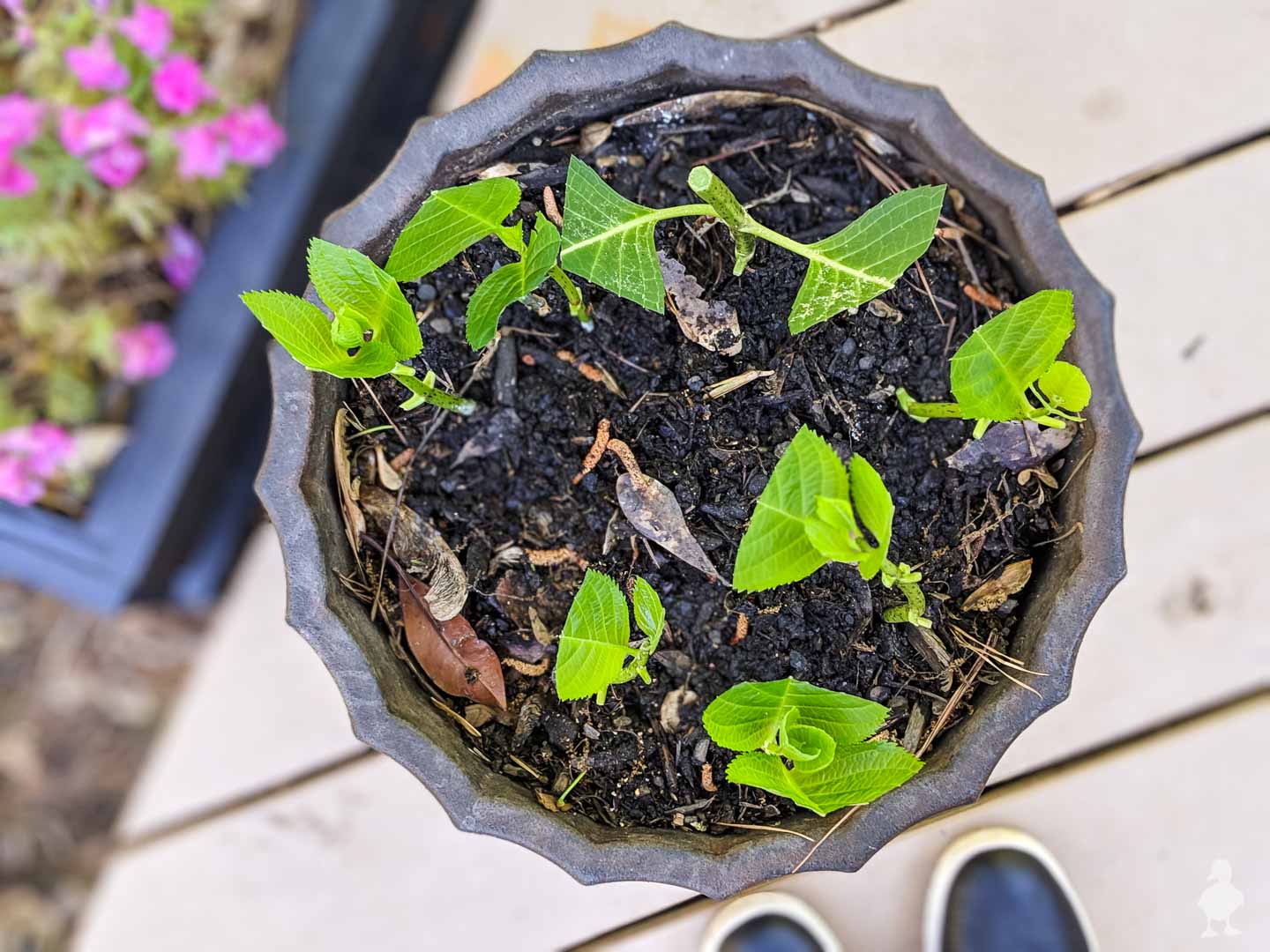The photograph is a horizontally aligned, rectangular image featuring a garden scene. Dominating the foreground, taking up about half of the frame, is an intricately designed iron or gray plastic flower pot with a scalloped, ridge-point edge, forming roughly 18 distinct points. The pot contains a mix of black soil, compost, and possibly broken-down wood chips, appearing dark and recently watered. Within the soil, there is evidence of a chopped-off stem, suggesting a larger plant has been cut down, along with several green leaves, some of which appear to be freshly severed and abruptly end with visible vein patterns.

Surrounding the main plant are three smaller plants on the lower right, also exhibiting leaves that are partially chopped off, with new foliage emerging. To the left of the central chopped stem, similar growth patterns are observed. Scattered within the pot are some brown leaves, likely blown in from elsewhere. The background of the photograph shows a white-painted wooden deck with horizontally aligned planks. To the right side, a pair of white-rimmed blue shoes are visible, hinting at the photographer's presence.

In the blurred background above and to the left of the main pot, there is a rectangular blue-painted wooden planter housing green leaves and pinkish-purple flowers. This aerial view captures the essence of a personal garden setup, possibly from a time shortly after the advent of color photography.